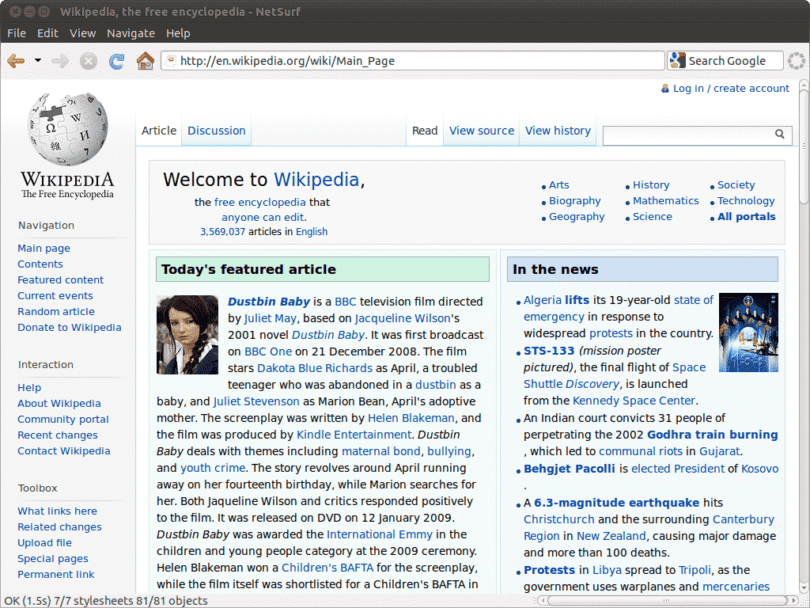This image showcases a screenshot of a Wikipedia page, slightly longer than it is tall. At the top, a horizontal black bar features essential controls including minimize, maximize, and close buttons, alongside the text "Wikipedia, the free encyclopedia" and the browser name "NetSurf." Below this bar is a toolbar containing menu options such as File, Edit, View, Navigate, and Help.

To the right of these menus, a gray border houses the Wikipedia search bar, additional icons, and the main page link. A Google search bar is positioned towards the right. On the left side, a vertical sidebar displays the Wikipedia logo and navigation options, including sections like Navigation, Interaction, and Toolbox, each containing several links.

Beneath the toolbar and sidebar lies a horizontally-oriented gray box with the text "Welcome to Wikipedia," offering various selectable categories. The main content area is divided into two columns. The left column, marked by a green header titled "Today's Featured Article," highlights an article on "Dustbin Baby" accompanied by an image. The right column features a blue header labeled "In the News," presenting a couple of recent news stories for the reader to stay updated.